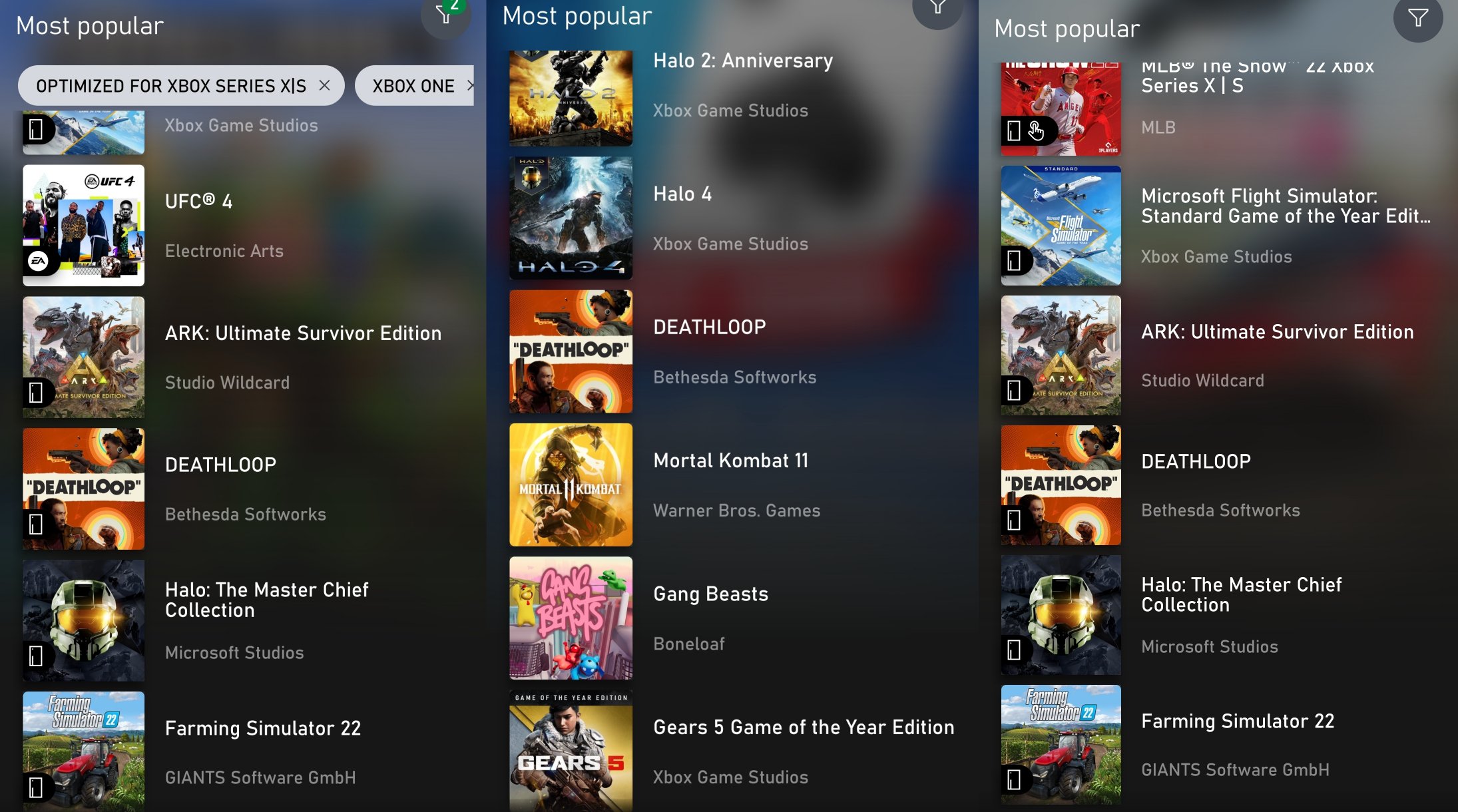Here are three distinct screenshots possibly taken from the Xbox mobile app. Each image features a blurry background with a mix of white and black tones, and a consistent label at the top left in white text reading "Most Popular."

In the first screenshot, there are icons that are light blue with rounded square shapes, labeled with text in black indicating "Optimized for Xbox Series X/S." Another visible label reads "Xbox One." This screenshot lists several game titles: "UFC 4," "ARK: Ultimate Survivor Edition," "Deathloop," "Halo Master Chief Collection," and "Farming Simulator 2022."

The second screenshot continues the list of popular games with titles: "Halo 2 Anniversary," "Halo 4," "Deathloop," "Mortal Kombat 11," "Gang Beasts," "Gears 5: Game of the Year Edition," and "MLB The Show for Series X/S."

In the third screenshot, there are repeated game titles, such as "Microsoft Flight Simulator: Standard Game of the Year Edition," "ARK: Ultimate Survivor Guide," "Deathloop," "Halo Master Chief Collection," and "Farming Simulator 2022." These repetitions might be an error or emphasize particularly popular games. 

Each game title is accompanied by a vibrant screenshot bursting with colors like reds, whites, blues, yellows, and greens, showcasing the dynamic visuals of the games featured in the Xbox mobile app.